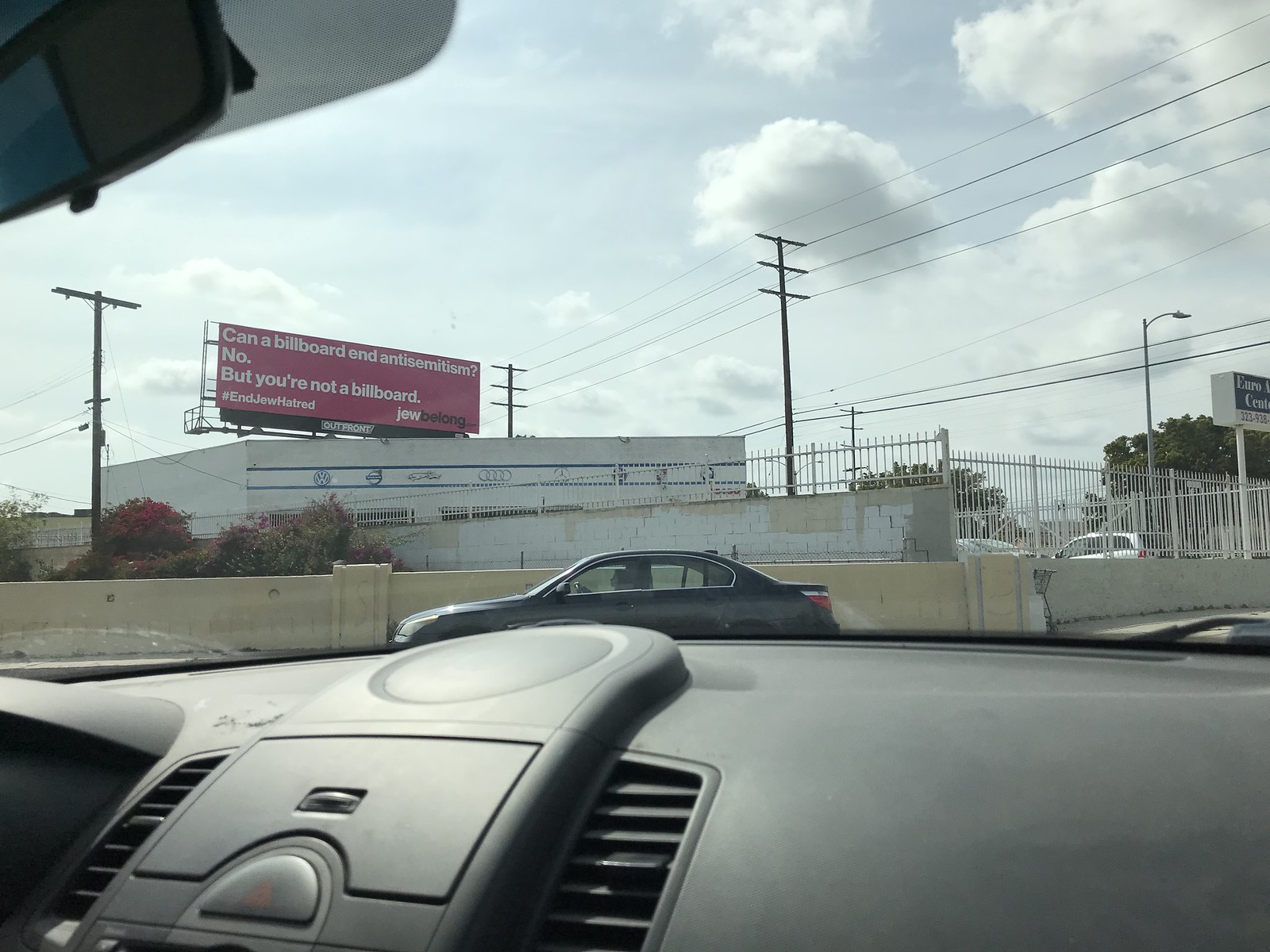The image captures the scene from inside a car, detailing the car's black dashboard, air vents, rear-view mirror, and part of the central console. Outside the window, a bright sunny day is evident, with a blue sky dotted with white clouds. Directly in front, a black car is seen making a turn at an intersection. The view includes a street divider and a brick wall painted partly in white and partly in cement color. Across the street, a white fence and another wall precede a building believed to be a car dealership, identifiable by the car logos and an array of cars in the lot. Scattered telephone poles, power lines, and street lamps add to the urban setting. Dominating the background is a red billboard with white text, reading: "Can a billboard end antisemitism? No, but you are not a billboard. #EndJewHatred." To the right of the billboard, another sign with white and dark blue colors is visible. Trees are sparse, completing the composition of this everyday urban snapshot.